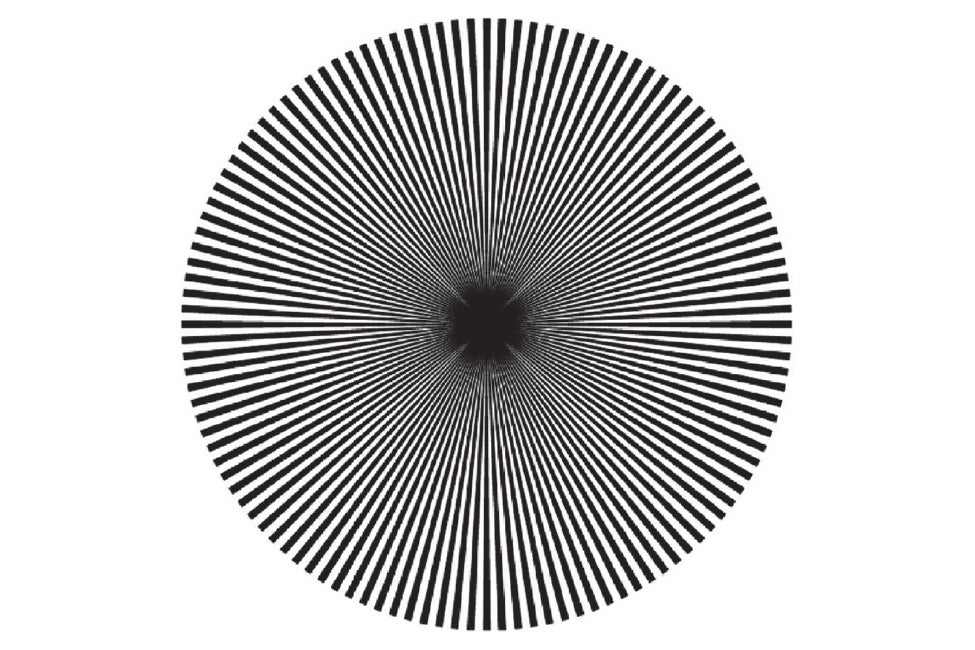This black-and-white image is a captivating optical illusion featuring a circular pattern that evokes the sense of peering into an abyss. The design consists of long, skinny triangles, reminiscent of needles or toothpicks, converging towards a very dark black center. These converging lines create a moiré pattern, causing your eyes to perceive movement and depth. The lines divide the image into four quadrants with a slight whiteness in the center area, enhancing the illusion of being drawn into a central void. The overall effect is similar to viewing the top of a wide vase that narrows sharply towards the bottom, or a floral, sunburst pattern that both bursts outward and caves inward depending on your perspective. This mesmerizing image distorts perception, making the center appear to enlarge and move as you gaze at it, and moves even more dynamically if you shift your head back and forth.